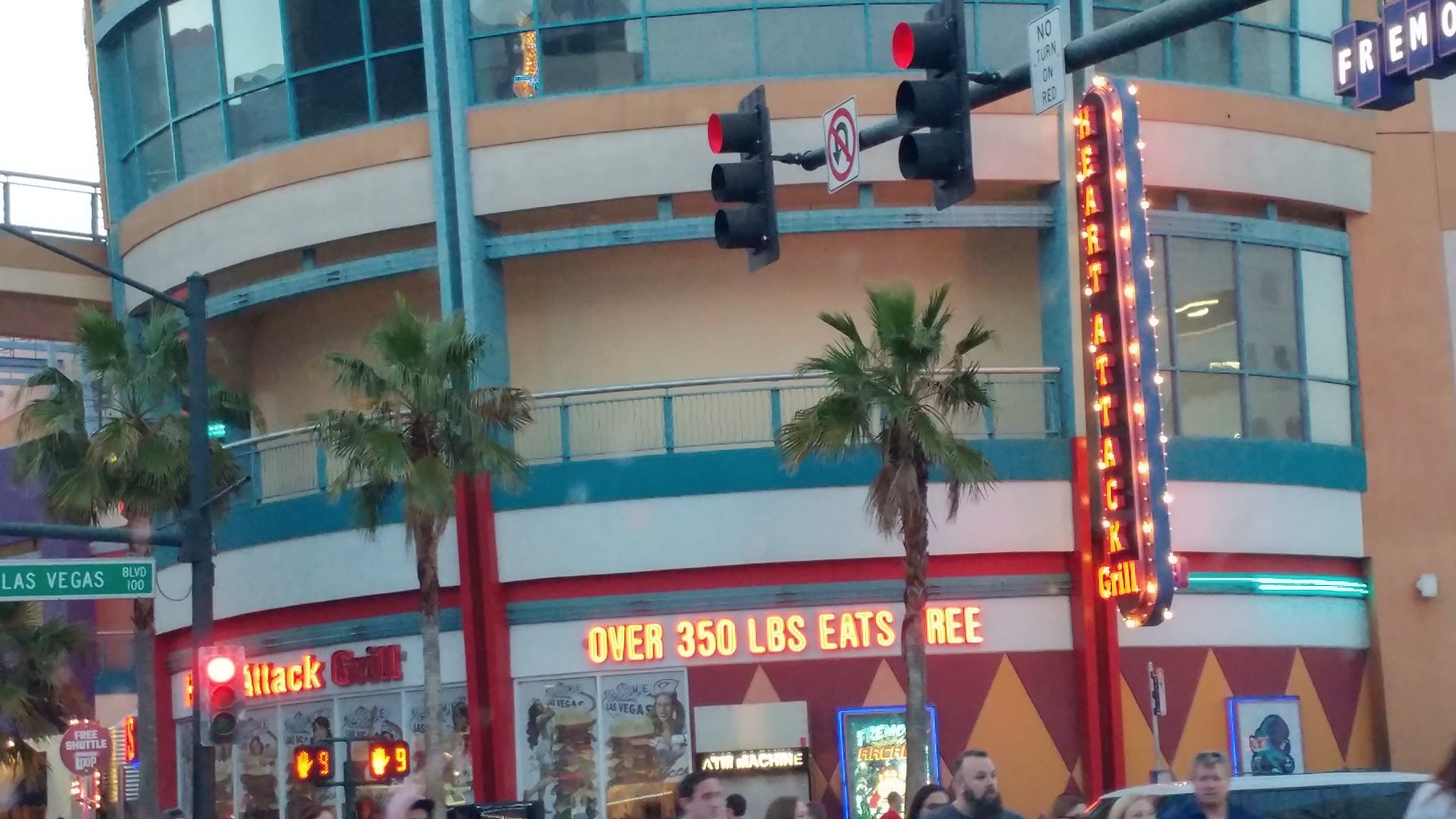The image captures a lively street corner on Las Vegas Boulevard featuring the iconic Heart Attack Grill. To the left, attached to a green streetlight pole, a green street sign marked "Las Vegas Boulevard 100" stands out. The same pole supports a glowing red traffic light. Dominating the scene is the Heart Attack Grill, known for its provocative marketing and controversial theme. The building has a distinct red, orange, and white exterior, emblazoned with a bright vertical neon sign reading "Over 350 pounds eat free," though a palm tree slightly obscures the word "free." The facade includes triangular design elements and window displays featuring images of nurses in revealing outfits holding oversized hamburgers. Additional signage includes a notification for a free shuttle and an ATM machine. In the background, you can partially see a movie poster-like sign. Palm trees punctuate the scene, their green leaves and brown trunks standing out against the urban backdrop. A few people's heads are visible at the bottom of the image, suggesting they are crossing the street, where a pedestrian signal indicates nine seconds remaining to cross. The bright and bustling atmosphere is quintessential of the Las Vegas experience.